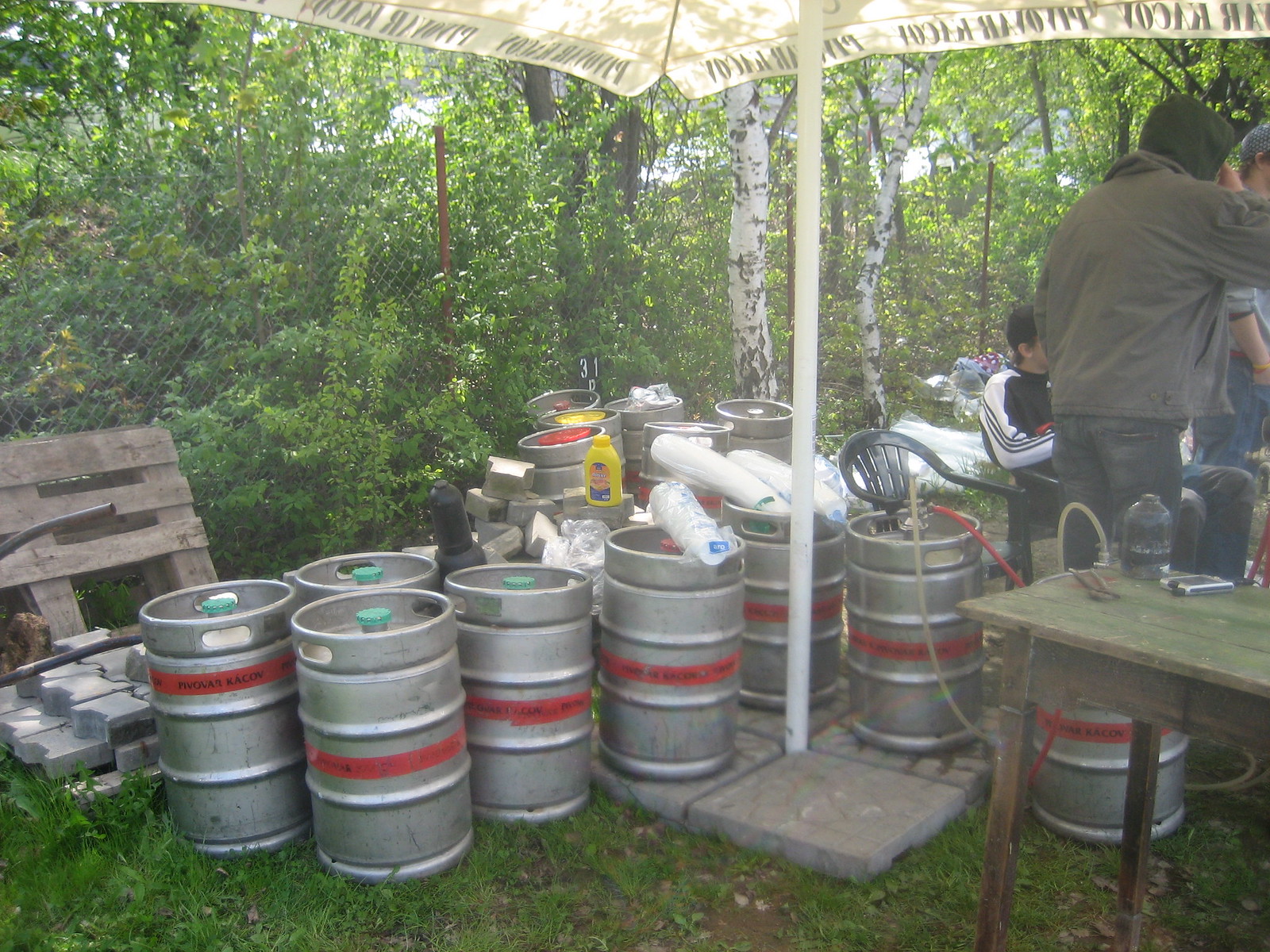In this outdoor photograph taken in a green, wooded area, a canopy supported by a single white pole covers roughly a dozen silver beer kegs, each adorned with a red stripe and featuring two handles on the sides. The pole stands on four concrete paving stones, with cups and possibly some tubing atop several kegs. Prominently in the lower right corner is a small wooden table with various objects on it. Two men stand to the right; one in a brown jacket with a black hood and black pants, the other in a dark shirt with blue jeans and his hand in his pocket. In the background, two black plastic lawn chairs support another person wearing a gray, black, and white shirt. The entire scene exudes a casual, backyard gathering ambiance.